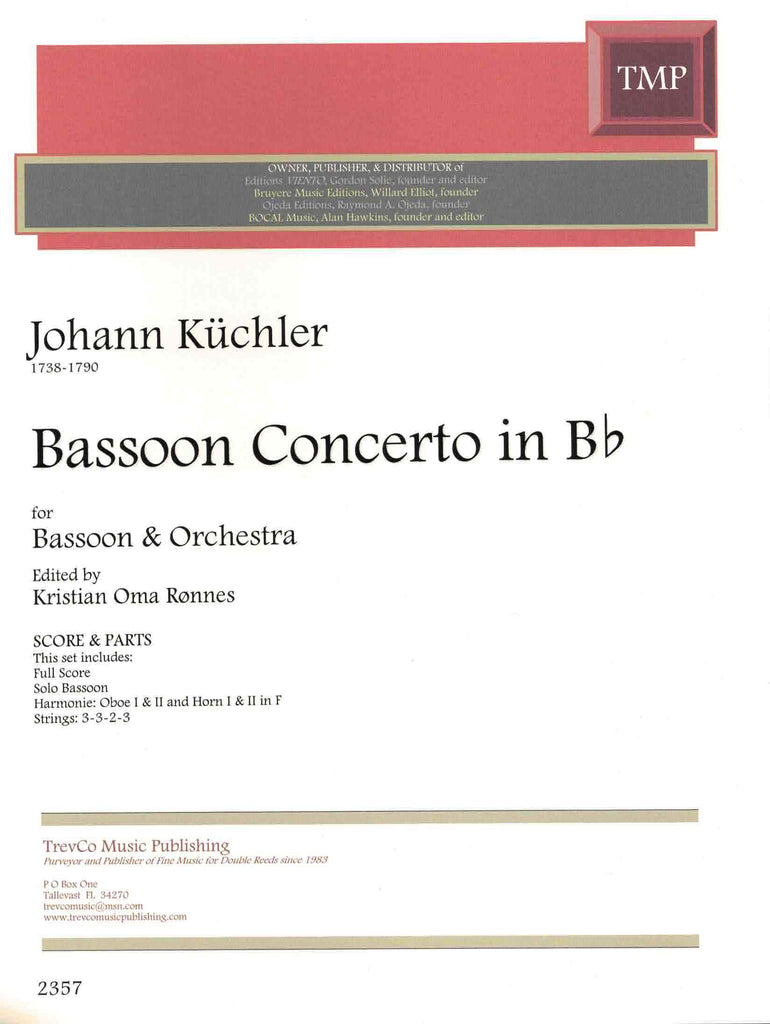The image depicts a detailed and colorful brochure for a concert by Johann Küchler, showcasing his life span of 1738-1790. At the top, a prominent pink bar with a logo reading "TMP" in a white square can be observed on the top right. Below it, there's blurred gray text. The central part of the brochure highlights "Johann Küchler" with the dates "1738-1790" underneath. The main piece of text emphasizes "Bassoon Concerto in B-flat for Bassoon and Orchestra," which has been edited by Christian Orner Rons, with details indicating it includes the score and parts. The lower section of the brochure bears the name "Trevco Music Publishing" along with their address. Additional information includes the set's contents, featuring a full score and solo bassoon parts, albeit in unclear text. Notably, the number "2357" is printed in black text at the bottom left corner.